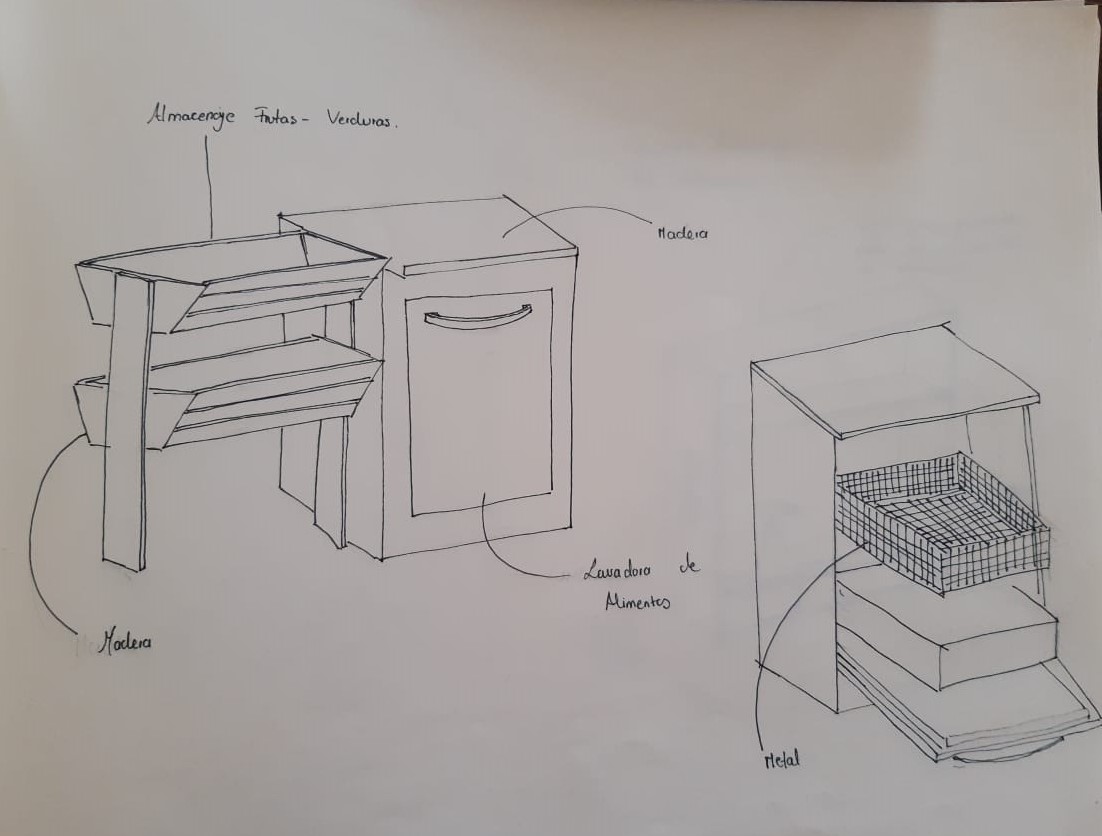This is a detailed photograph showcasing a series of hand-drawn furniture designs on a white sheet of paper. Each piece of furniture is meticulously illustrated and accompanied by black cursive annotations. 

The first drawing depicts a unique piece with two basket-like structures positioned at the top, supported by legs on either side. Adjacent to this, a cabinet is sketched, featuring a circular handle spanning its front and a flat top surface.

To the side, another detailed drawing illustrates a multi-level drawer unit. It comprises three distinct pull-out sections: one adorned with lines, another plain, and the third displaying a complex, layered design. This unit also boasts a flat top. 

The artistic sketches are visually striking, providing a clear view of the various furniture concepts, each annotated for clarity.